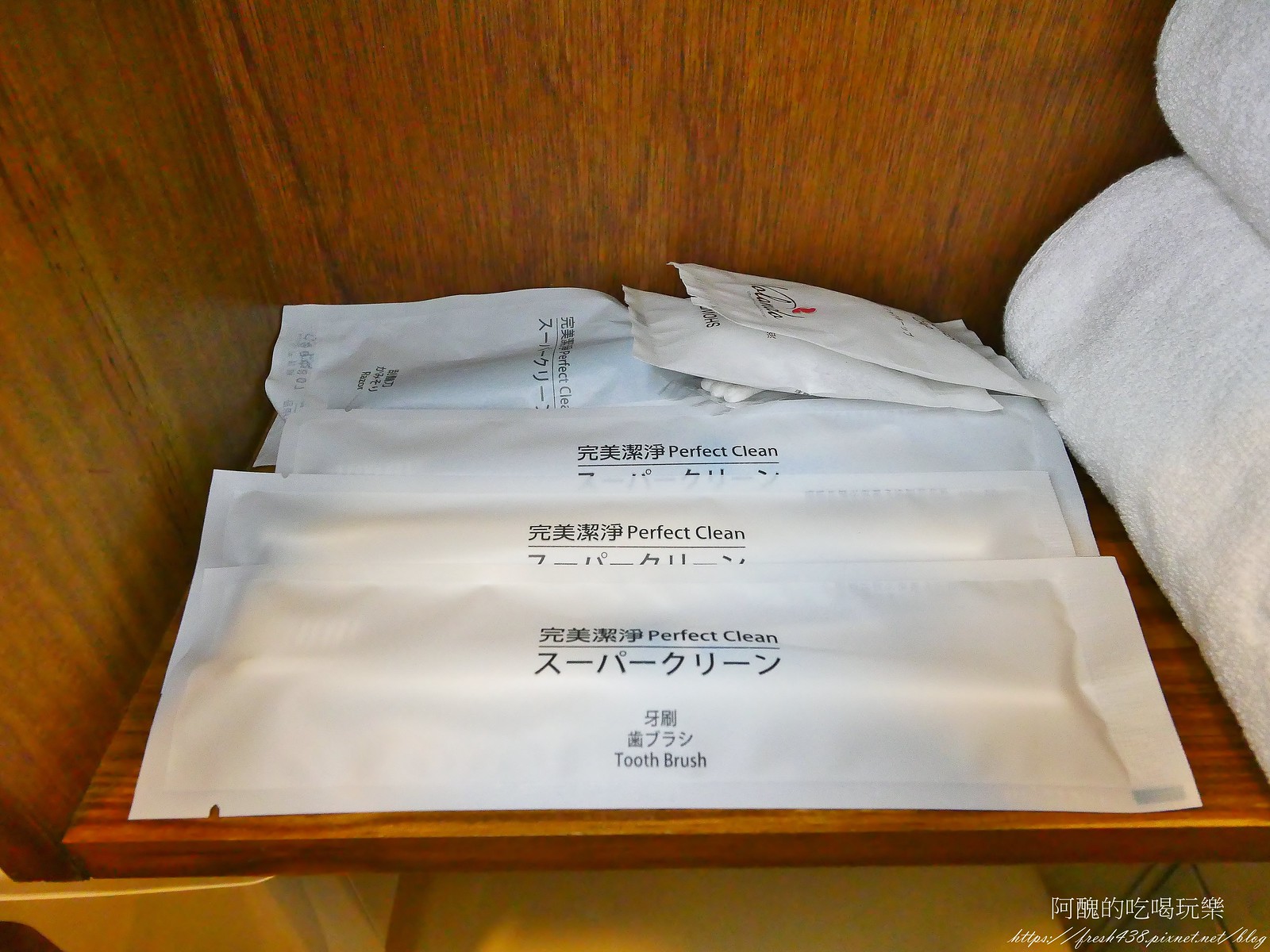The image depicts the interior of a wooden shelf, likely found in a hotel or guesthouse, possibly of Asian origin. On the right side of the shelf, two white towels are neatly rolled up and placed, reminiscent of typical hotel presentation. In the central and left sections of the shelf, there are several individually packaged items intended for personal use. The most prominent of these items are three white plastic packets labeled "Perfect Clean Toothbrush" in both English and Asian characters, likely Japanese, Chinese, or Korean. Additionally, there are other smaller packets towards the back, which might contain toiletries such as soap or dental floss, although their exact contents are unclear. The shelf itself appears to be made of wood, possibly teak, and sits above a yellow item or surface, which might be an orange bin or envelopes, adding a splash of color to the scene. The overall setup suggests a neat and organized provision of amenities commonly found in hotel bathrooms.